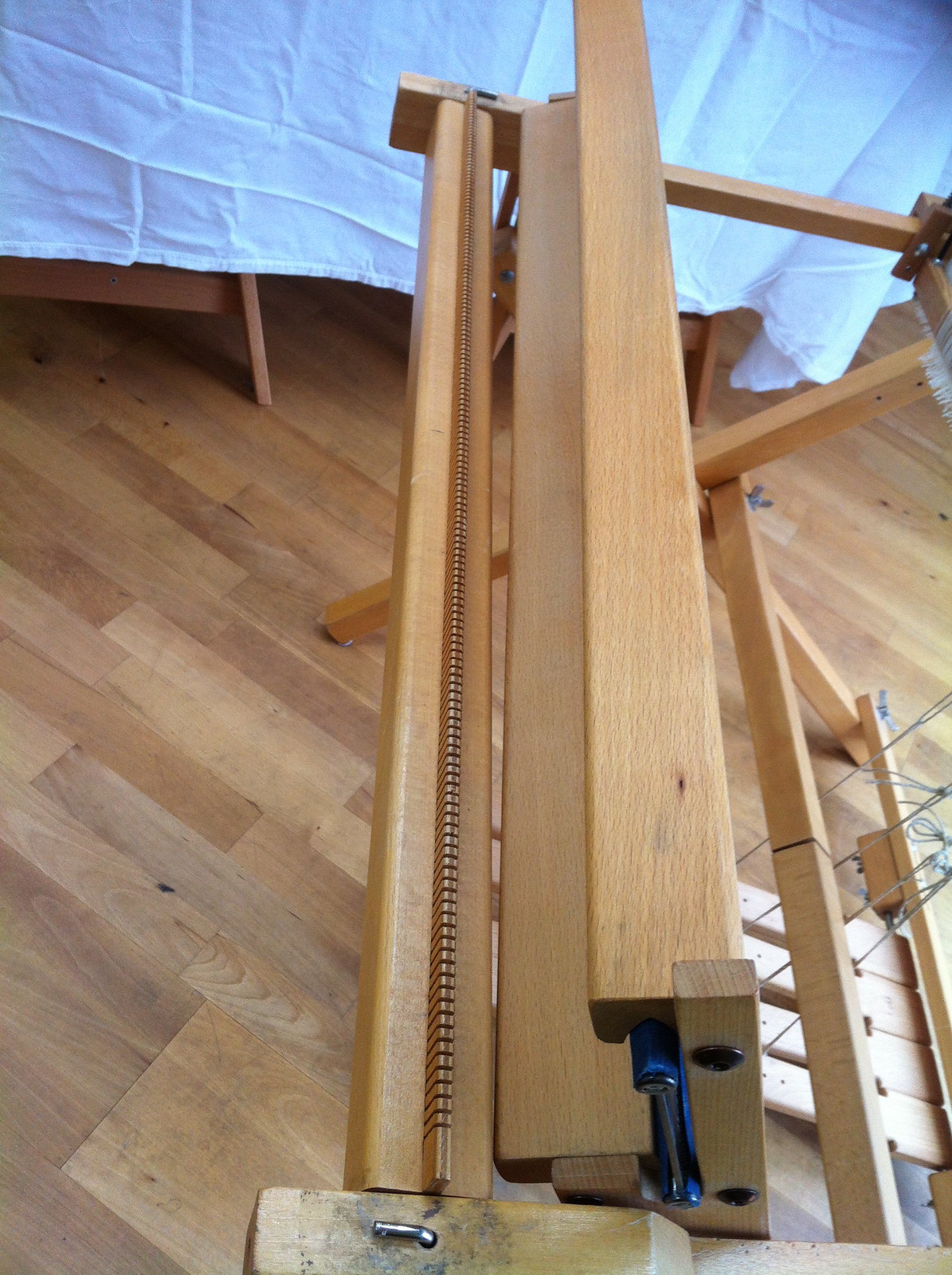The photograph captures a wooden loom, meticulously crafted from light-colored wood and evidently designed for weaving fabrics. Though currently devoid of thread or fabric, it features wooden foot pedals with attached retention strings. This loom appears lightly used and well-maintained, hinting at either a modern recreation or a refurbished piece, as modern hardware, including screws and wing nut washers on its legs, indicate an updated design. Positioned on a hardwood floor, the loom is set against a backdrop where more wooden structures can be partially seen, draped under a white sheet. A general work area can also be discerned, suggesting the early stages of a woodworking or fabric project, with cloths visible on a table in the background.